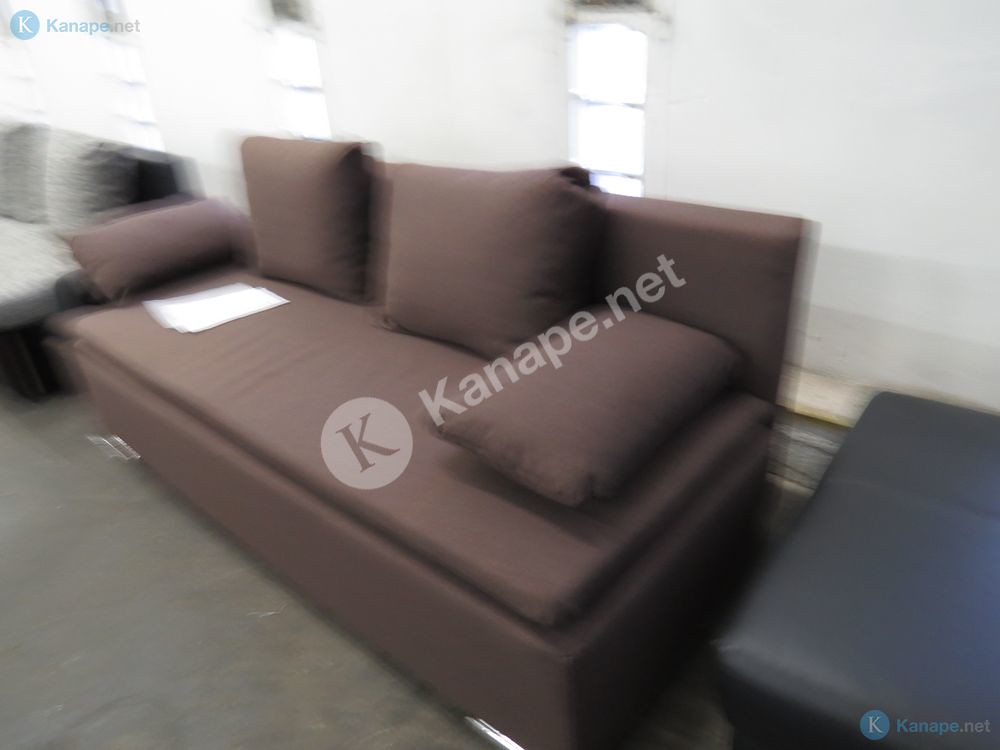This blurry color photograph depicts a brown couch positioned against a white wall in a room with three windows. The design of the couch is quite angular, featuring a rectangular base with a flat, rectangular cushion on top. It has no armrests and silver feet at the bottom. The seating area includes four cushions: three larger, pillowy ones, and one smaller horizontal cushion. A brown pillow is placed on the left end of the couch, while one cushion is laying down on the right end. Scattered on the couch are some white pieces of paper. In the background, partial views of a white couch to the left and a black leather ottoman or similar piece of furniture to the right can be seen. The image also features a watermark of K-A-N-A-P-E dot net with a K logo, appearing twice: one in blue font with a circle in the top left corner, and another in brown diagonally across the middle.